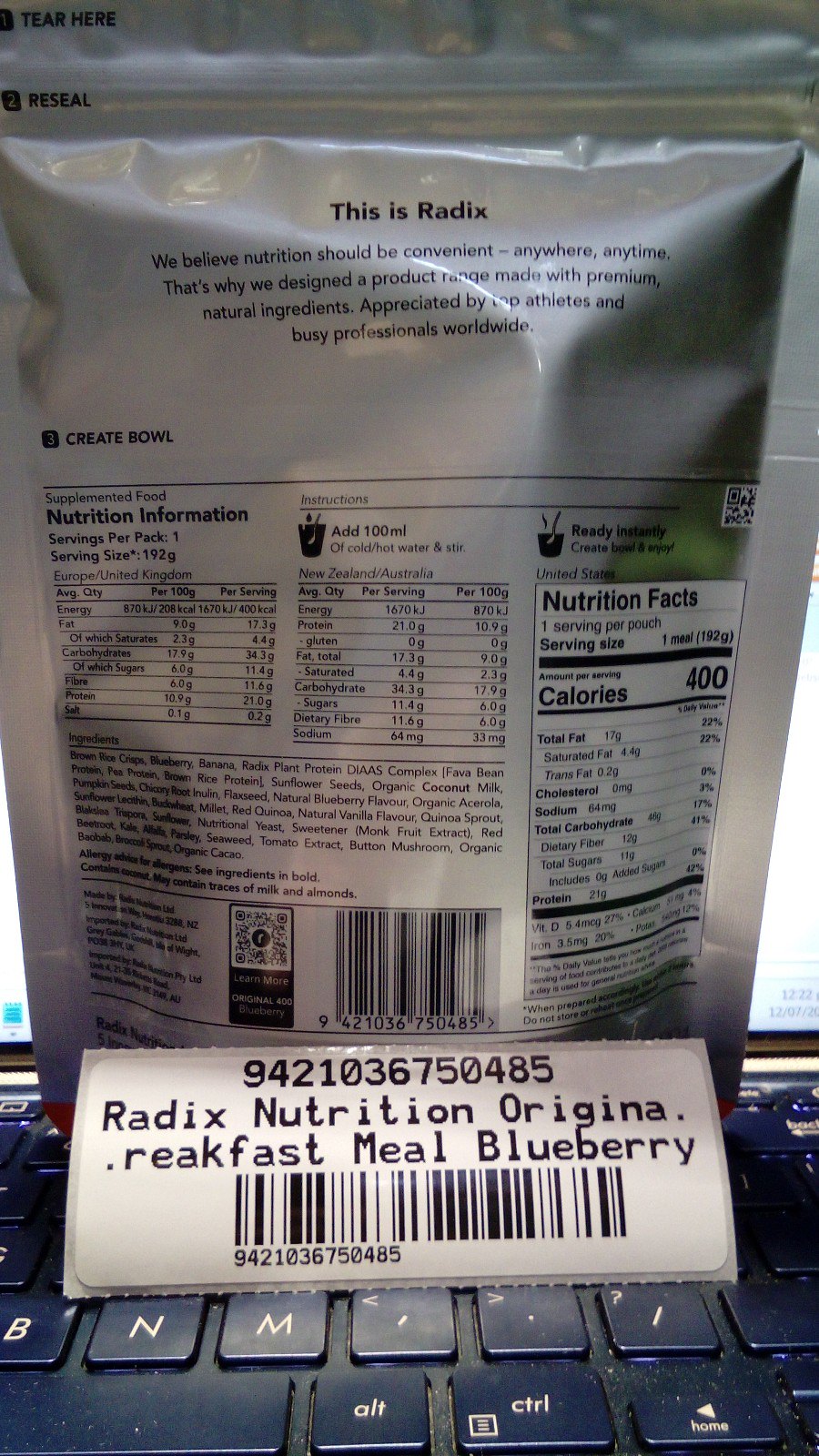The image showcases the back of a standing, upright bag of Radix Nutrition Powder, specifically the Original Breakfast Meal in a blueberry flavor. The bag is made of gray plastic and features a comprehensive label. This label includes detailed nutritional information, a thorough list of ingredients, and a breakdown of proteins and nutrients presented in three different formats. A barcode is prominently displayed at the top of the label. In the foreground, the bottom two rows of a keyboard are visible, suggesting the bag is placed atop or near a keyboard, with a sticker bearing a barcode partially resting on the keyboard. The label also features the brand's ethos, stating: "This is Radix. We believe nutrition should be convenient anywhere, anytime. That's why we designed a product range made with premium natural ingredients appreciated by top athletes and busy professionals worldwide."